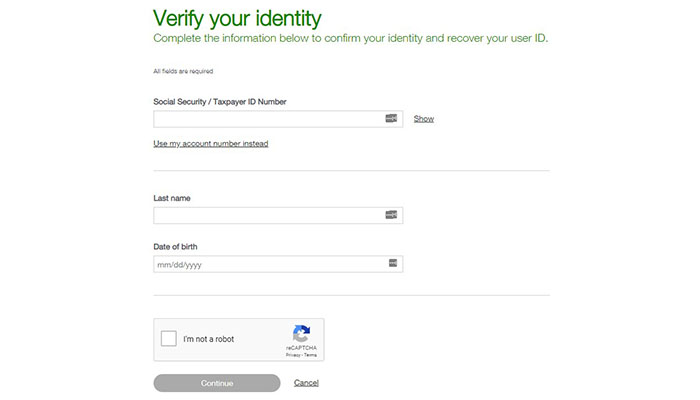The image showcases a web page displaying a personal information verification form. The predominant background color is white, with green text at the top. The main heading reads "Verify Your Identity" and is followed by a subheading in smaller green text that states, "Complete the information below to confirm your identity and recover your user ID."

Just below this, there's a small note in black text saying "All fields are required." The form begins with a section labeled "Social Security/Taxpayer ID Number" with a blank field to fill in. Beneath this section, there is an option in underlined black text reading "Use my account number instead."

A thin, light gray line separates this section from the next, which prompts the user to fill in their "Last Name" in black text, followed by an empty field for the input. Further down, the form asks for the "Date of Birth," with a placeholder format "MM/DD/YYYY" in a smaller text field.

Another thin gray line separates these fields from the verification section at the bottom. Here, a gray rectangle contains a white check box labeled "I'm not a robot." Next to this is the reCAPTCHA icon, which features three arrows in a circle colored gray, blue, and dark blue, with the label "reCAPTCHA." 

At the bottom left corner, there is a gray button with the text "Continue" in white font, with an underlined "Cancel" option next to it.